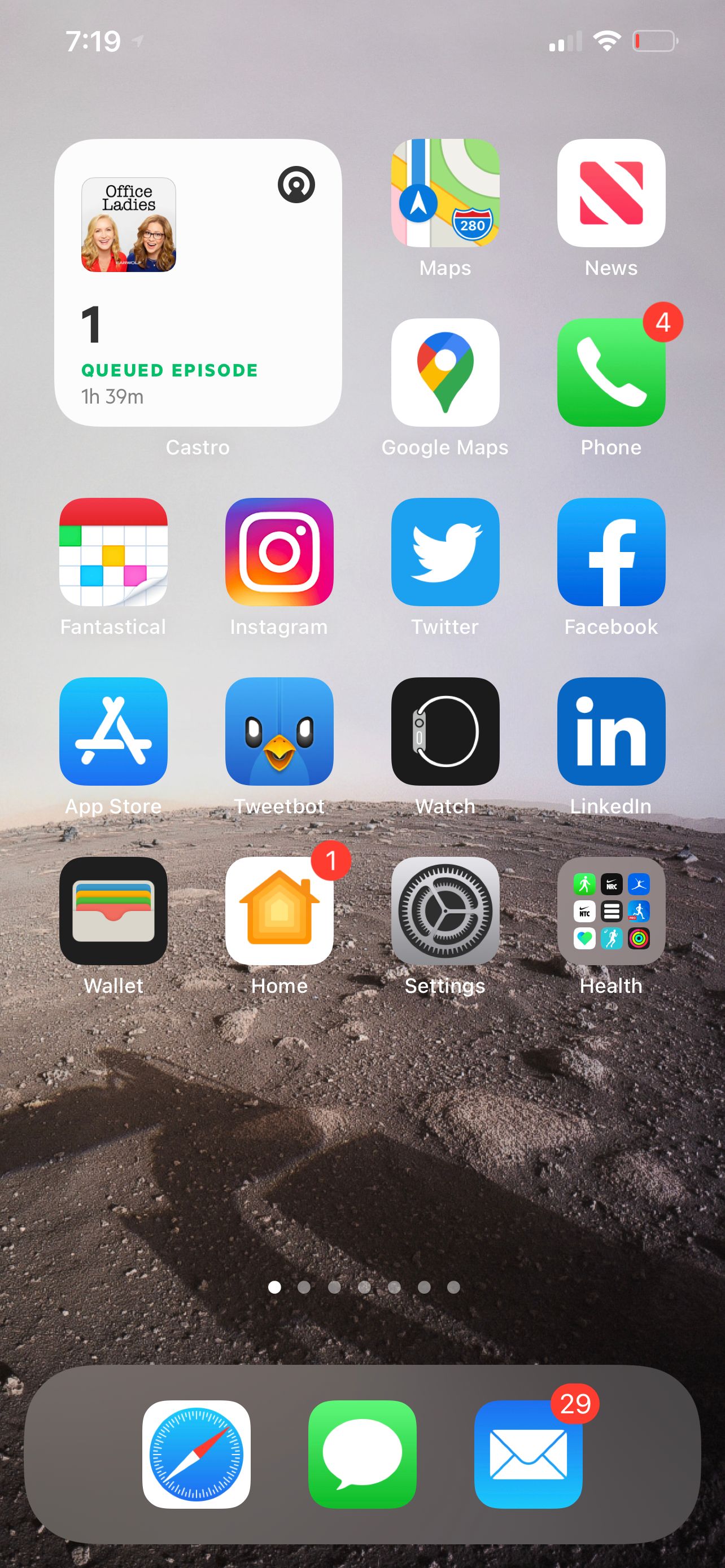A phone screenshot displays the main page of a device, featuring a background image that could be interpreted as the Moon landing, a beach scene, or the surface of Mars. The time shown is 7:19, with a two-bar signal strength, activated Wi-Fi, and a critically low battery at approximately 10%. The top left indicates "Office Ladies," queued up at 1 hour and 39 minutes on the Castro app, suggesting the user was watching an episode.

The main page showcases a variety of apps, including Maps, News, Google Maps, and the Phone app, which reveals four missed calls or messages. Other visible apps are Fantastical, Instagram, Twitter, Facebook, App Store, Tweetbot, Watch, LinkedIn (criticized as a less favorable version of Facebook), Wallet with a notification badge, Home (also with a notification badge), Settings, and Health. The bottom section shows an email icon with 29 unread messages. Additionally, there is a chat box icon and a built-in compass.

Several more app pages are accessible, indicated by the presence of multiple dots for swiping left or right.